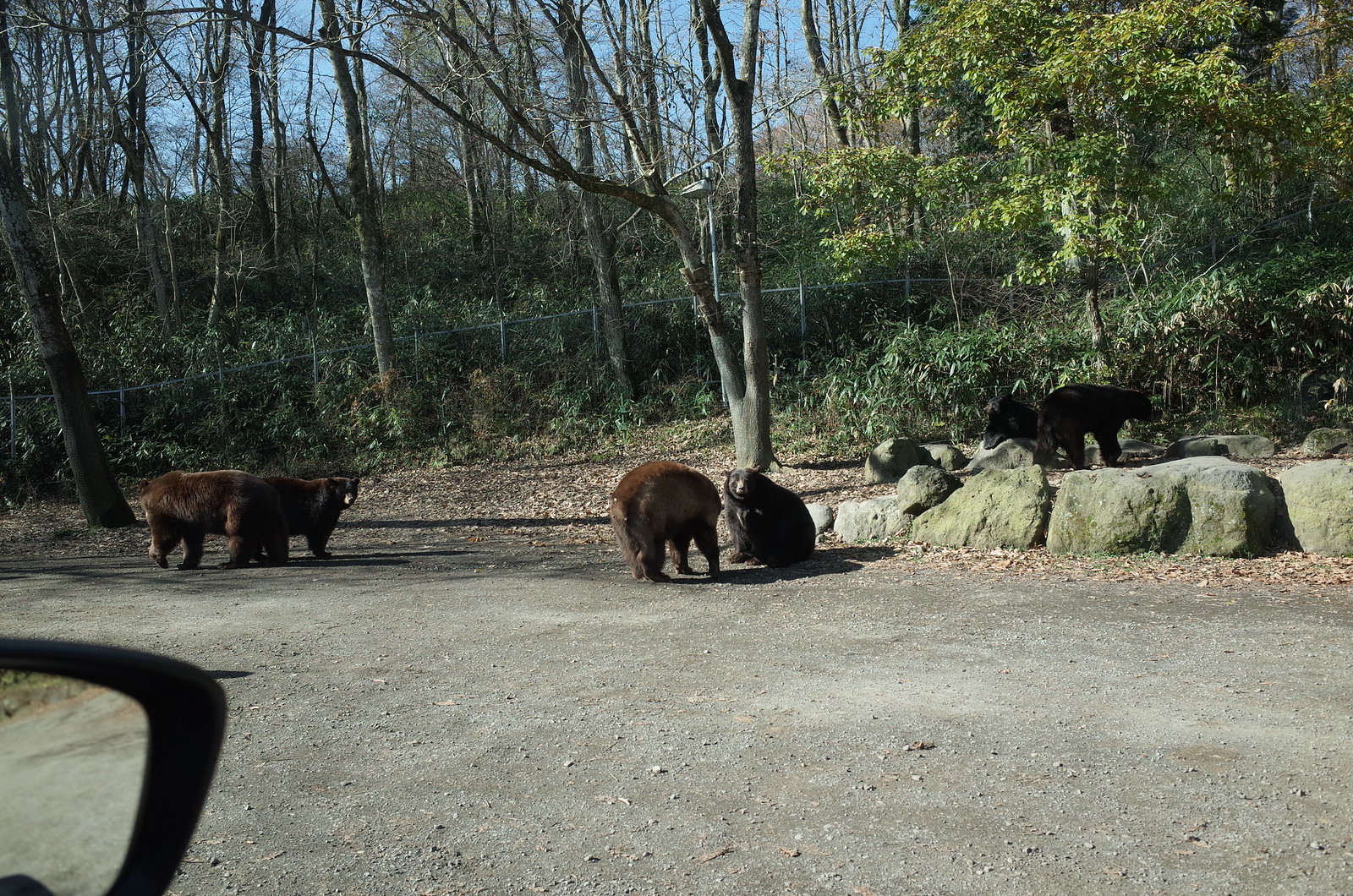The image depicts a zoo enclosure with a dirt floor scattered with leaves and moss-covered rocks. The enclosure houses five bears, an even mix of brown and black, with most bears visible in small groups or pairs, either lounging or meandering about. In the background, there is a gray chain-link fence, beyond which a hill covered in bushes, shrubbery, and additional slender trees extends upwards. These trees, both inside and outside the enclosure, are not particularly tall or thick, creating a sparse, almost transitional forest vibe, possibly indicating early spring or autumn. The image also captures a partial view of what seems to be a car's side view mirror in the left-hand corner, suggesting it was taken from within a vehicle.